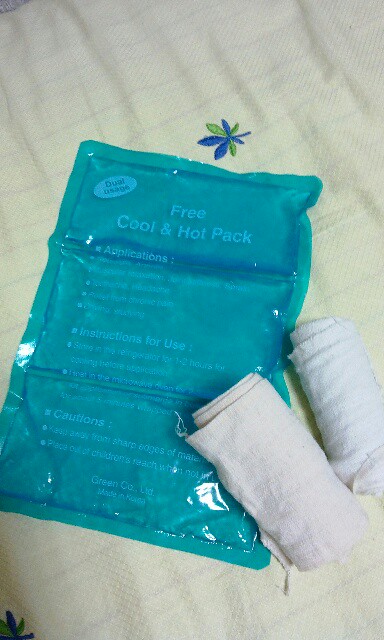In this portrait-mode image, the focus is a free dual-usage cool and hot pack of an aqua blue color, prominently positioned in the center. The pack, appearing smooth and gel-like, is divided into three foldable sections. The top section displays the words "Free Cool and Hot Pack," while instructions and application information span the top and middle sections, with caution notes on the bottom section. The background is primarily a white cloth or bedspread, adorned with an embroidered flower consisting of blue and green stalks, near the top area. The hot and cool pack lies on this spread, flanked by two white rolled-up gauze pads on its side and partially on top, suggesting a hospital or therapeutic setting for pain relief, likely after an injury or sprain.